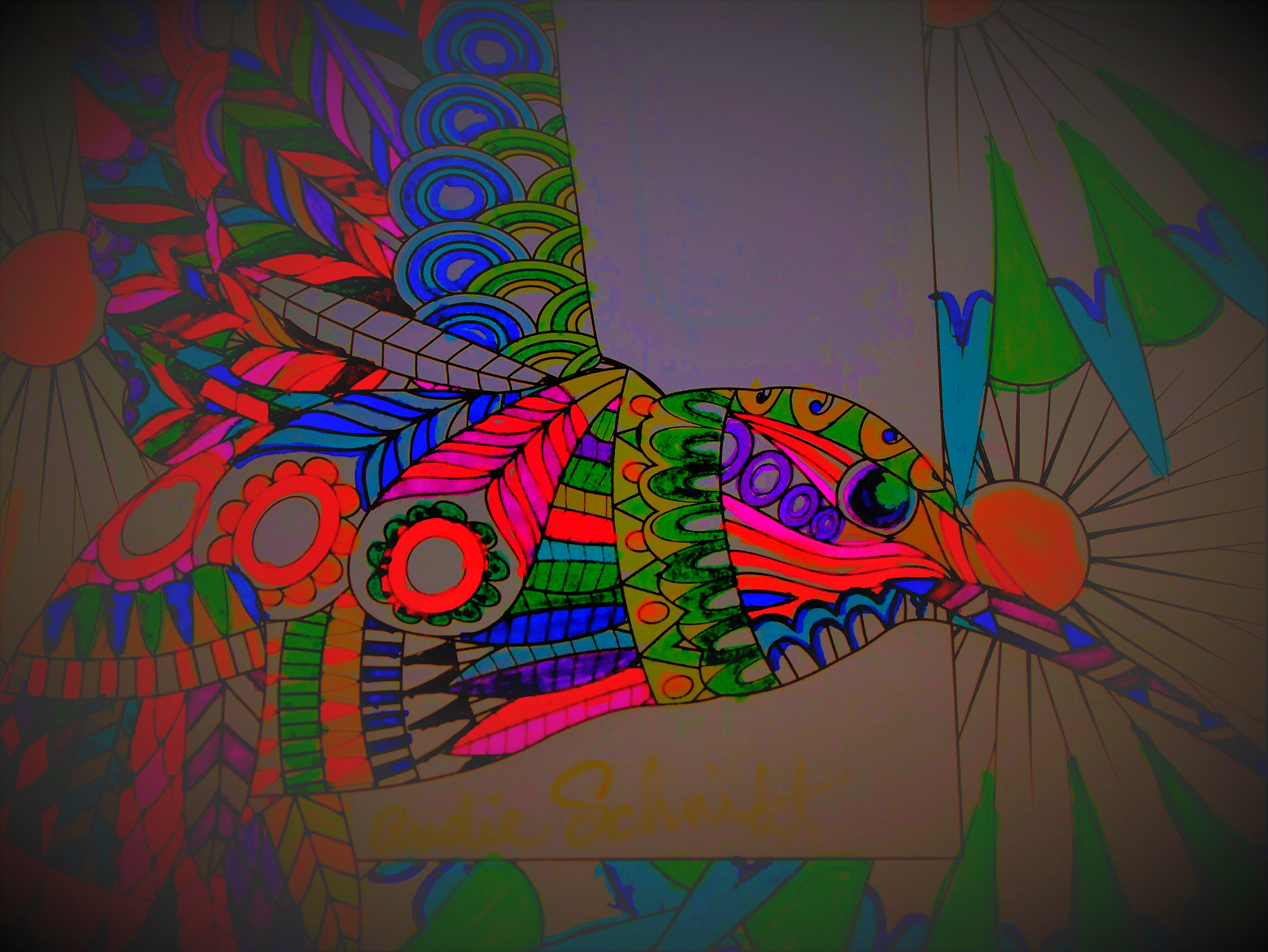This color photograph captures a complex and visually intriguing piece of art. The artwork evokes the aesthetic of stained glass but with more abstract elements and forms. At first glance, it appears to be a depiction of a bird or possibly an insect, characterized by its roundish head oriented to the right. The head features what seems to be a distinct beak and wings that extend upward and backward.

The figure is composed of multiple bands of vibrant colors including red, green, blue, pink, and a purplish hue. Within these bands, intricate patterns such as circles, flowers, and lines resembling feathers are interwoven, enhancing the stained glass effect. The beak area is particularly striking, featuring a red round hump embellished with radiating black rays.

In the upper and lower corners of the image, there are intersecting green and blue triangles with distinctive dips, adding another layer of geometric complexity. The background transitions from a dark grey at the top to a more brownish tone at the bottom, providing a stark contrast to the vivid colors of the central figure.

Beneath the bird, there appears to be a signature written in dark yellow ink, although it is too dim to decipher clearly. The entire composition is rich in detail and depth, inviting the viewer to explore its many facets and interpretations.